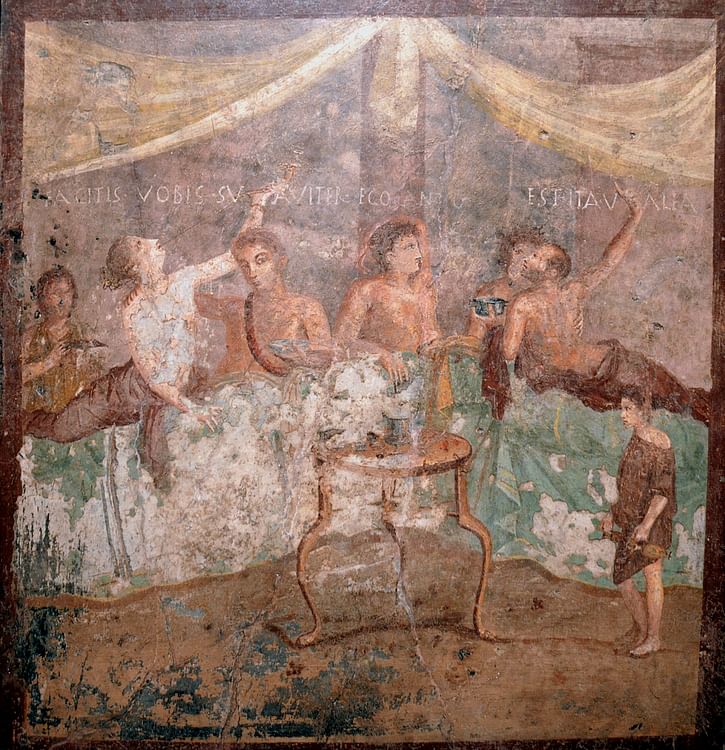This wall painting, rendered in muted hues of browns, blues, and mauves, portrays a classic banquet scene reminiscent of ancient Greek or Roman culture. Central to the composition is a white table with delicate, ornate legs, around which several individuals are gathered, reclining and engaging in a communal feast. The participants, possibly four men and three women, are partially covered by a grand tent-like canopy that drapes over a prominent post in the background. Latin or ancient Greek script adorns the upper portion of the painting, adding to the historical ambiance. Notably, one figure, possibly a slave, stands to the right, dressed in tattered clothing, highlighting the social dynamics of the era. The image exhibits visible signs of age, with some areas, particularly around the ambiguous figure on the right, showing paint degradation.